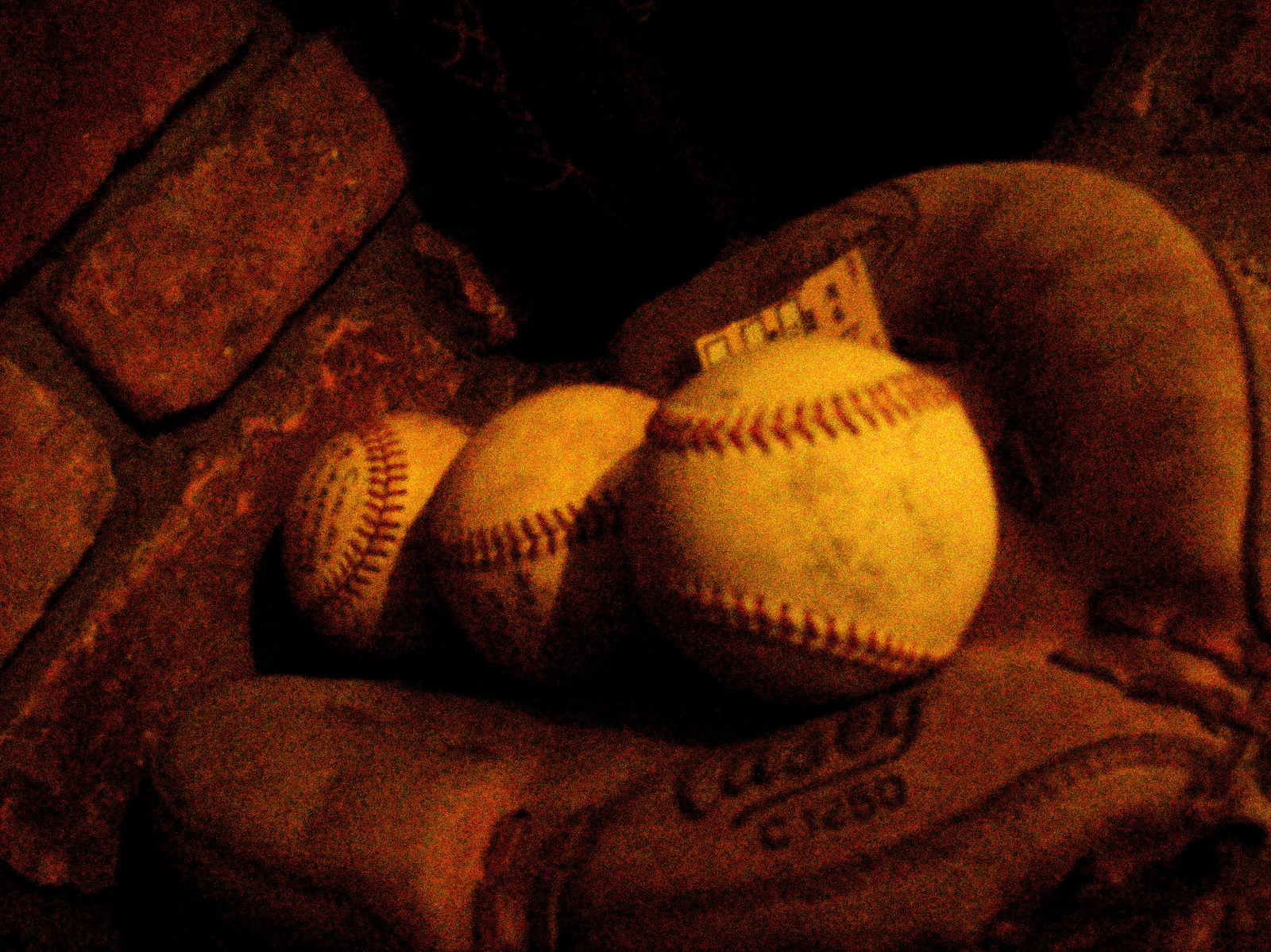The photo appears to be a grainy nighttime shot taken outdoors, capturing an older style catcher's mitt on a brick fireplace mantel with visible mortar. The deep red brick wall frames the left side of the image. The well-worn brown leather glove, labeled "Casey" in cursive with "C 1250" beneath it, dominates the center. Nestled into its palm are three baseballs, which appear tan due to the brown color scheme of the photo. The baseballs, featuring red chevron stitching, also display some black writing. A small yellow card with white squares and tiny writing sticks out from behind the rightmost baseball. The overall image has a sepia-like tone, emphasizing earthy browns from dark to light.